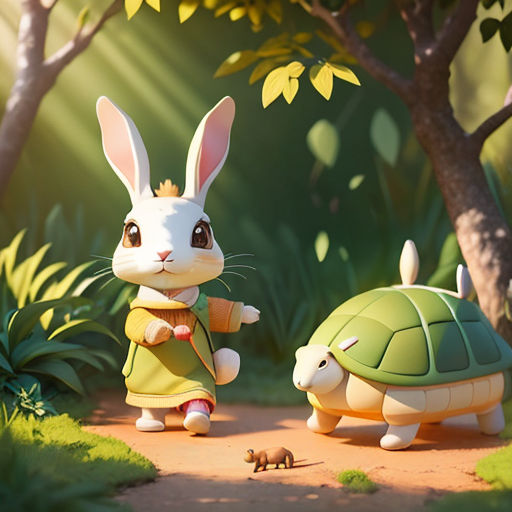The image depicts a vibrant, hand-drawn cartoon scene set in a lush forest. On the right-hand side stands a tall tree with green leaves, mirrored by another tree in the distance on the left side. The forest floor is adorned with green foliage and grass. In the foreground, a dirt trail runs through the scene. On the right side of the path is a small turtle with a green shell and white legs. To the left of the trail, a well-groomed rabbit walks on two feet, dressed in a colorful green jacket. Both animals are attentively gazing at a small, mysterious brown creature positioned between them. This tiny critter, difficult to identify, stands in the middle of the trail, adding an element of curiosity to the whimsical woodland tableau.